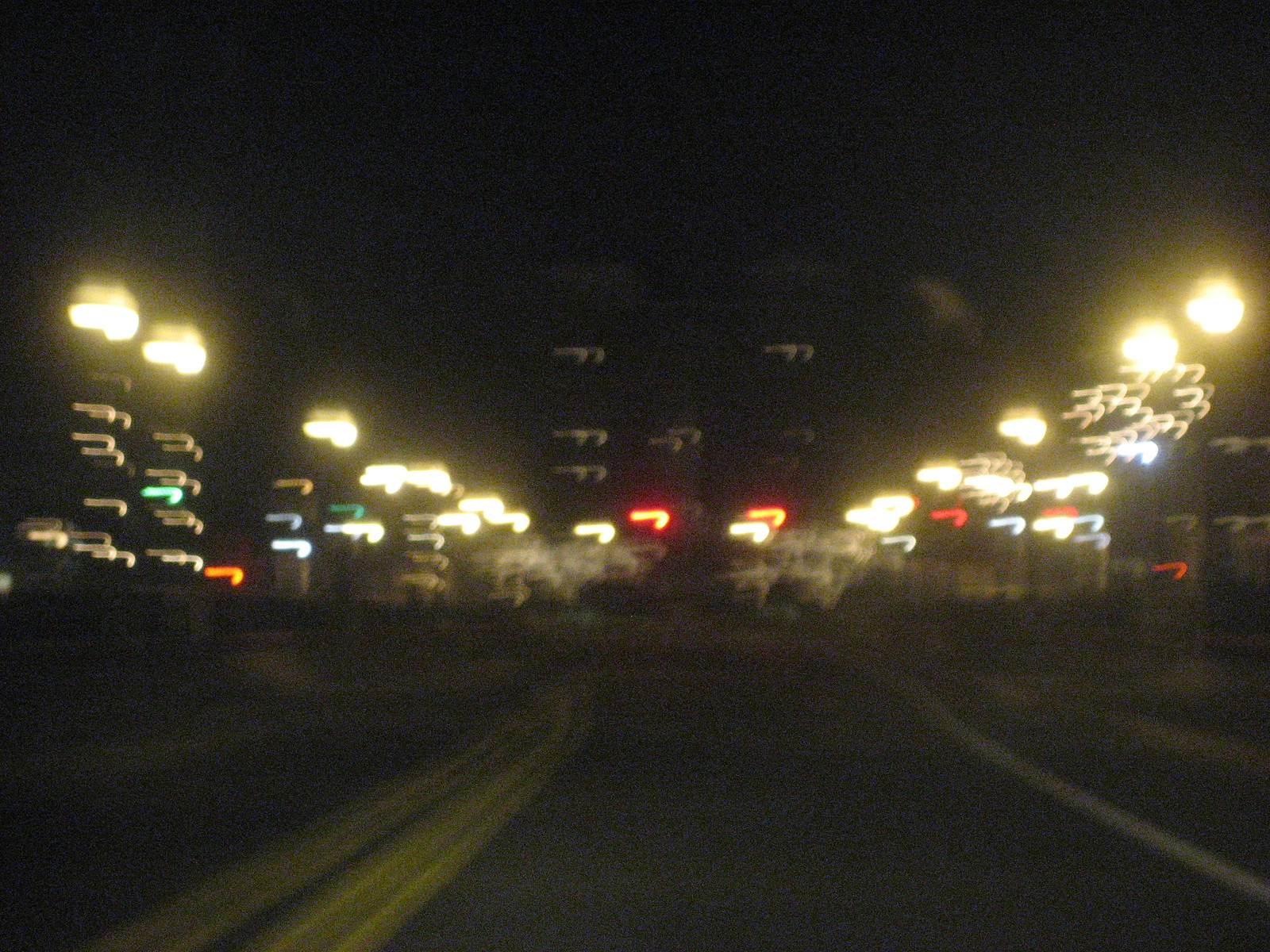A nighttime cityscape photograph captures a dreamy, almost surreal scene viewed from the front windshield of a moving vehicle. The top portion of the image is a pitch-black sky, emphasizing the late hour. In the foreground, the asphalt road features a series of white and yellow lines, which are blurred into multiple overlapping streaks due to the motion. This gives the impression of parallel lanes running chaotically into the distance.

Street lamps line both sides of the road, their lights stretching into distorted, glowing orbs. The nearest lamp on the right side appears to have twin globes atop its post, though the exact details are fuzzy. The lamps further along the road meld into blurry lines and shapes, punctuating the scene with warm, glowing spots that trail off into the night.

Further embellishing the photograph are blurred neon lights from distant buildings. These lights are smeared into shapes resembling hooked staples or candy canes lying on their sides. The colors range from white and orange to blue, yellow, and green, creating a vibrant, almost chaotic palette that lights up the road.

In the distant background, two blurry structures stand out—possibly towers, buildings, or the uprights of a bridge—partially illuminated by or reflecting various city lights. Their indistinct forms add to the overall haze and mystery of the scene, capturing the frenetic energy and dazzling confusion of a city at night.